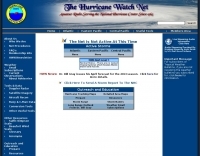This image appears to be a screenshot of a website, though it is incredibly blurry, making most of the text unreadable except for the main headline and the website’s name. The layout, however, can be described in detail:

At the top of the page, there's a dark blue header about two inches tall, with almost blackish shades on the left and right edges. Approximately an inch below this, the page transitions to a blue segment on both the left and right sides, with a white background filling the central area.

In the top left corner, there's a bordered yellow box containing some text and bisected by a horizontal line. The upper portion of this box is light blue while the lower part is dark blue. In the grey middle section, the top line features the words "The Hurricane Watch Net" in blue lettering. Below this, there's red text that is too blurry to read clearly. Further down, a white space suggests a search bar area.

Under this, five sections span across the page. The left side of the page is densely packed with white text, while the right side has white text filling about half the column. In the white central portion, blue lettering stands out. Below this, there's a tab with a blue upper half and a grey lower half, filled with various writings that are hard to decipher.

Continuing down, there’s a smaller tab with a light blue top section followed by blue and white areas, which also contains unreadable text. Below this, two lines of text are visible but not clear enough to be read. Another tab follows, starting with light blue at the top, transitioning to progressively darker shades of blue, and featuring black text throughout.